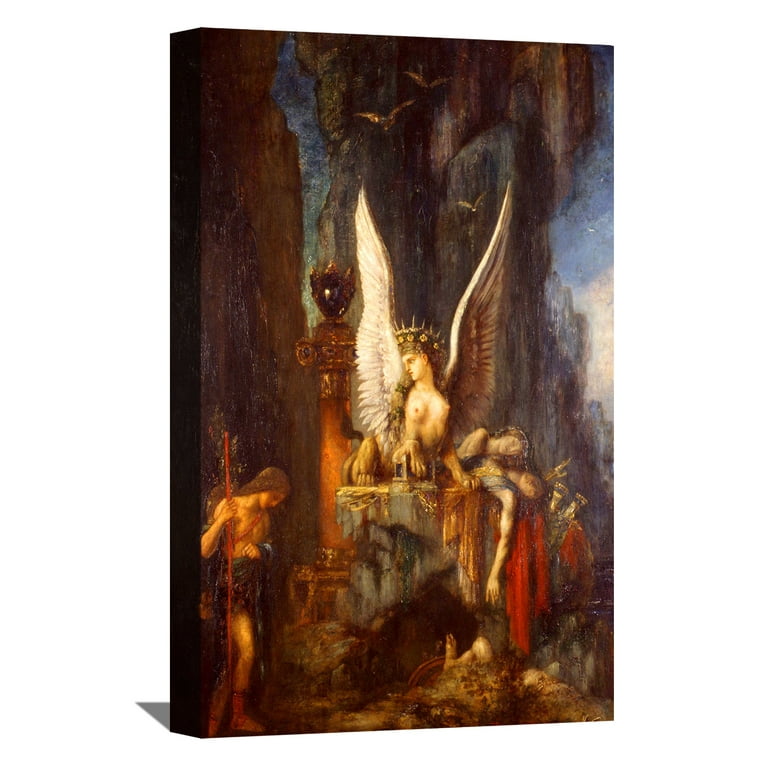The painting is a vertical rectangular oil painting on canvas, rich in dark, dramatic tones and religious or mythological symbolism. At its center is a prominent altar with two figures laid across it. One figure is a half-woman, half-eagle creature, featuring strikingly large, pointed white wings reminiscent of a pegasus or angel. She wears a king's crown and is nude from the waist up, displaying her bare breasts. Below the waist, she possesses the lion-like features of back legs and paws. 

Behind her wings, an eye-like shape is discernible in the shadowy background. Flanking the altar, a man clad only in a loincloth stands to the side, holding a spear and gazing downward. There is a woman in a long, red dress bending over the altar, with indistinct figures or objects clustered at her feet, partially obscured due to the darkness. Additionally, on the bottom left, another person stares at the ground while gripping a pole. 

To the painting's right side, a hallway leads to a slightly lighter area, suggesting the presence of a window. The enigmatic setting is further accented by birds, possibly resembling pterodactyls, flying overhead, and a column topped with a round blue sphere, enhancing the painting's otherworldly atmosphere.